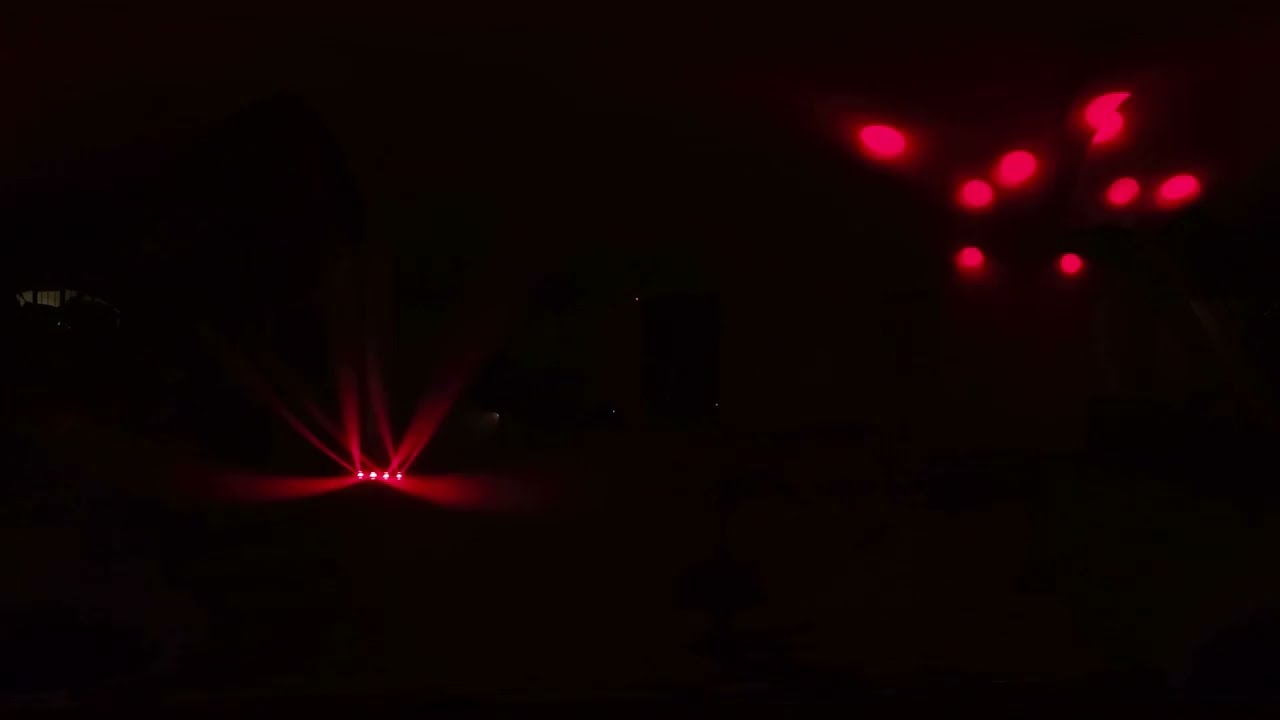The image, oriented in a 16 by 9 landscape, portrays a very dark, predominantly black background, suggesting it was taken at night. Throughout the darkness, vivid red lights punctuate the scene. In the lower left quadrant, a row of four intensely bright red lights emits light flares and beams that shoot upwards diagonally toward the top of the image. Additionally, in the center-left area, more red lights can be observed, adding to the scattered illumination. Dominating the upper right quadrant, there is a collection of eight red orbs, with one orb intriguingly appearing split or doubled. These red lights, reminiscent of tail lights or perhaps even the mysterious allure of spaceship lights, create a stark contrast against the dark backdrop, illuminating their surroundings and forming the primary visual elements in an otherwise minimalistic scene.